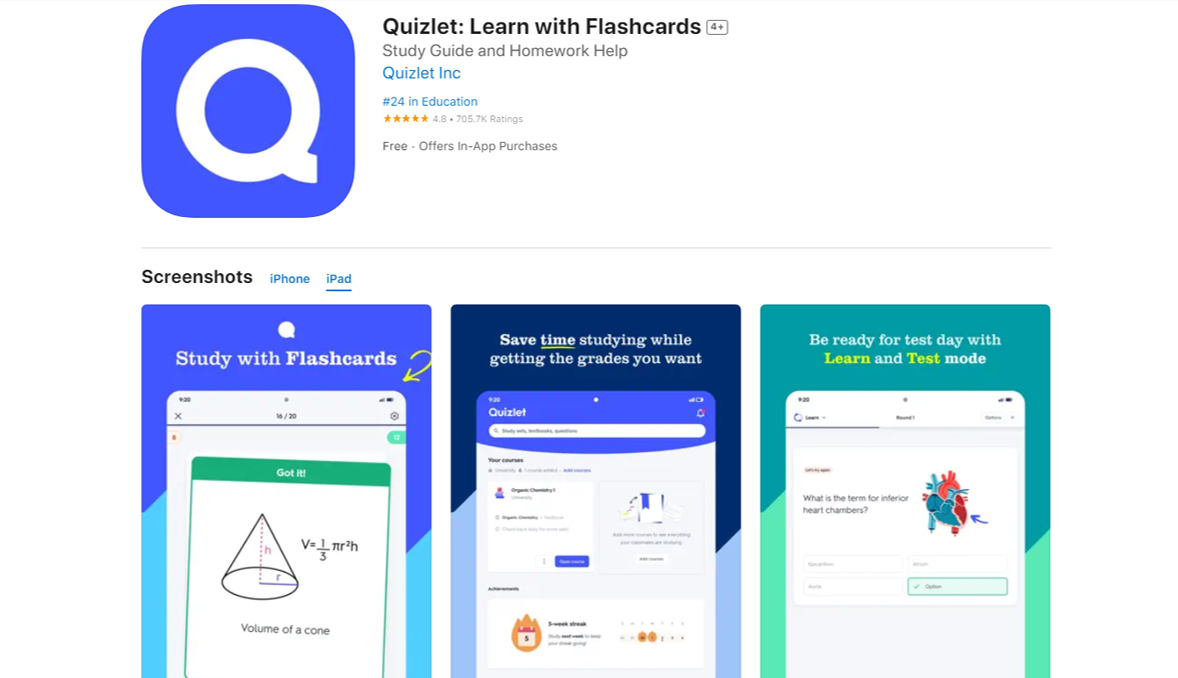This image captures a detailed screen display from the Quizlet app, specifically showcasing its "Learn with Flashcards" feature. Prominently featured is a large blue cube icon next to bold, black text that reads "Quizlet Learn with Flashcards." Below this, the text "Study Guide and Homework Help" appears alongside "Quizlet, Inc., number 24 in Education," signifying its ranking and function in the educational category. 

The app boasts a high rating of five stars with an overall score of 4.8. Adjacent to this rating is some faded red text, though the specific words are not clear. The app is noted to be "Free" but includes "offers in-app purchases."

Beneath this information is a section labeled "Screenshots," with examples suitable for both iPhone and iPad devices. The first screenshot illustrates a study flashcard featuring a cylindrical shape and the equation "V = 1/3," indicative of geometry-related content. Captions reiterate phrases like "Study with Flashcards."

In the center of the image, accompanying the text "Save Time Studying While Getting the Grades You Want," there is a small media image with the Quizlet logo, along with visible interface elements including a search bar and areas that likely track study progress, such as a daily streak.

Further details highlight the feature "Be Ready for Test Day with Learn and Test Mode," complemented by an icon resembling a heart. At the bottom, something is highlighted, but its contents are not fully visible. The entire composition underscores Quizlet's utility in providing effective study aids and resources to improve academic performance.